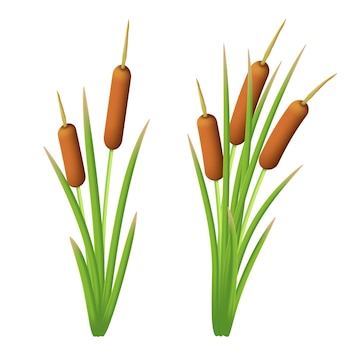The image depicts two cartoon-style illustrations of wild plants against a solid white background. Each plant features long, narrow, green blades of grass that fan outwards. Notably, both plants include unique hot dog-shaped structures, with each brown structure attached to the green stems. The plant on the left showcases two blades of grass and three of these brown cylindrical formations, one of which has a yellow point emerging from its top. The right plant displays three similar brown structures. These hot dog-like shapes are tan in color, transitioning from brown at the base to a lighter yellowish hue towards the top. The plants are depicted with no shadows, emphasizing their bold, simple cartoon aesthetic.